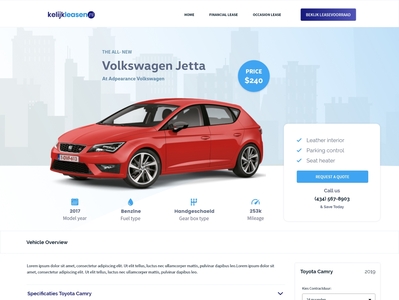**Screenshot of Volkswagen Site: New 2023 Volkswagen Jetta Advertisement**

This detailed screenshot showcases the Volkswagen website featuring the all-new 2023 Volkswagen Jetta. Dominating the image is a sharp, red Volkswagen Jetta set against a minimalist, silhouetted skyline graphic. The price, prominently displayed, is $240, potentially indicating a monthly lease rate.

At the top of the site, adjacent to the Volkswagen logo, are three text menu options and a large blue button for easy navigation. Below the Jetta image, four distinct sections with icons provide key information about the vehicle:

1. **Model Year:** Indicates "2023" as the model year.
2. **Engine Type:** Mentions "Benzine fuel type," confirming it uses petrol.
3. **Gearbox Type:** Features a graphic of a gearbox labeled "Handgeschakeld" (manual transmission) with five gears.
4. **Mileage:** Displays "25.3 K," likely referring to fuel efficiency of 25.3 kilometers per liter, with an accompanying mileage meter icon.

Additional features are listed with check marks, highlighting elements such as leather interior, parking control, and seat adjustments, alongside a prompt to "Request a Quote" accompanied by a displayed phone number.

Despite some references to a Toyota Camry, the focus remains on the impressive specifications and features of the 2023 Volkswagen Jetta, making it a compelling choice for prospective buyers.